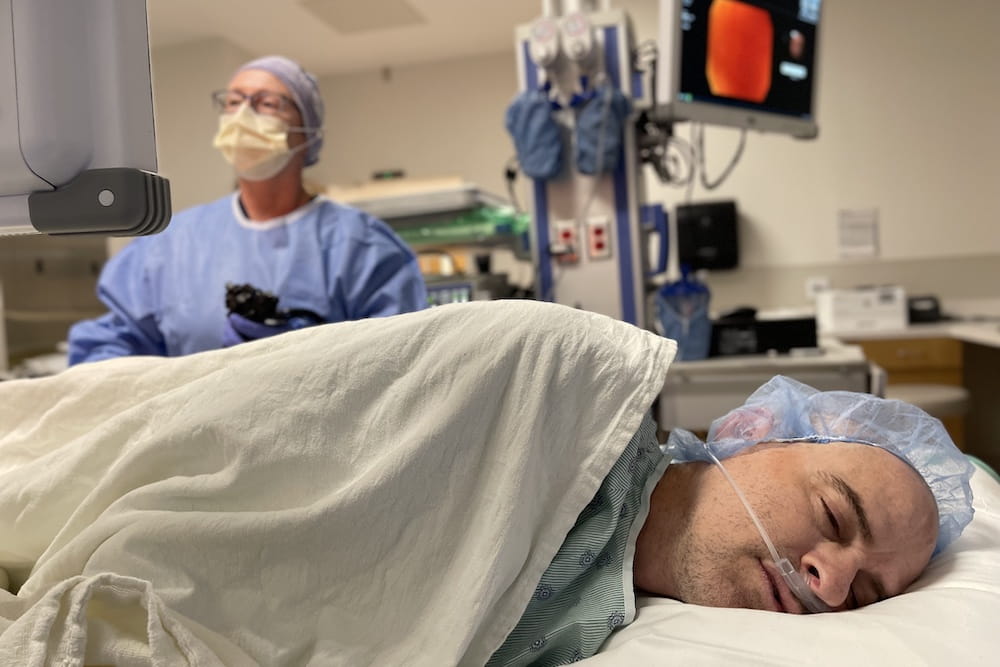The image depicts a detailed hospital setting where a male patient lies on a bed, facing the camera, in a surgical context. He is positioned on his right side with a light blue hair cap and grey stubble visible on his face. He's receiving oxygen through a nasal tube and is covered by a white sheet, partially revealing a blue gown. His eyes are closed, suggesting he is either asleep or sedated. 

In the background, a female medical technician, possibly a nurse, is seen standing and focused on a computer screen. She is dressed in typical surgical attire, including a blue gown, a face mask, glasses, and latex gloves. The nurse's hands are occupied with a black object, which isn't clearly identifiable. 

Surrounding the scene is an array of medical equipment, some clearly visible and other parts blurred. Various devices are connected to sockets with visible wiring, contributing to the clinical atmosphere. Notably, behind the patient's head, a monitor displays a black screen with a red square, amidst other equipment including a green and white unit, further emphasizing the medical environment's complexity.